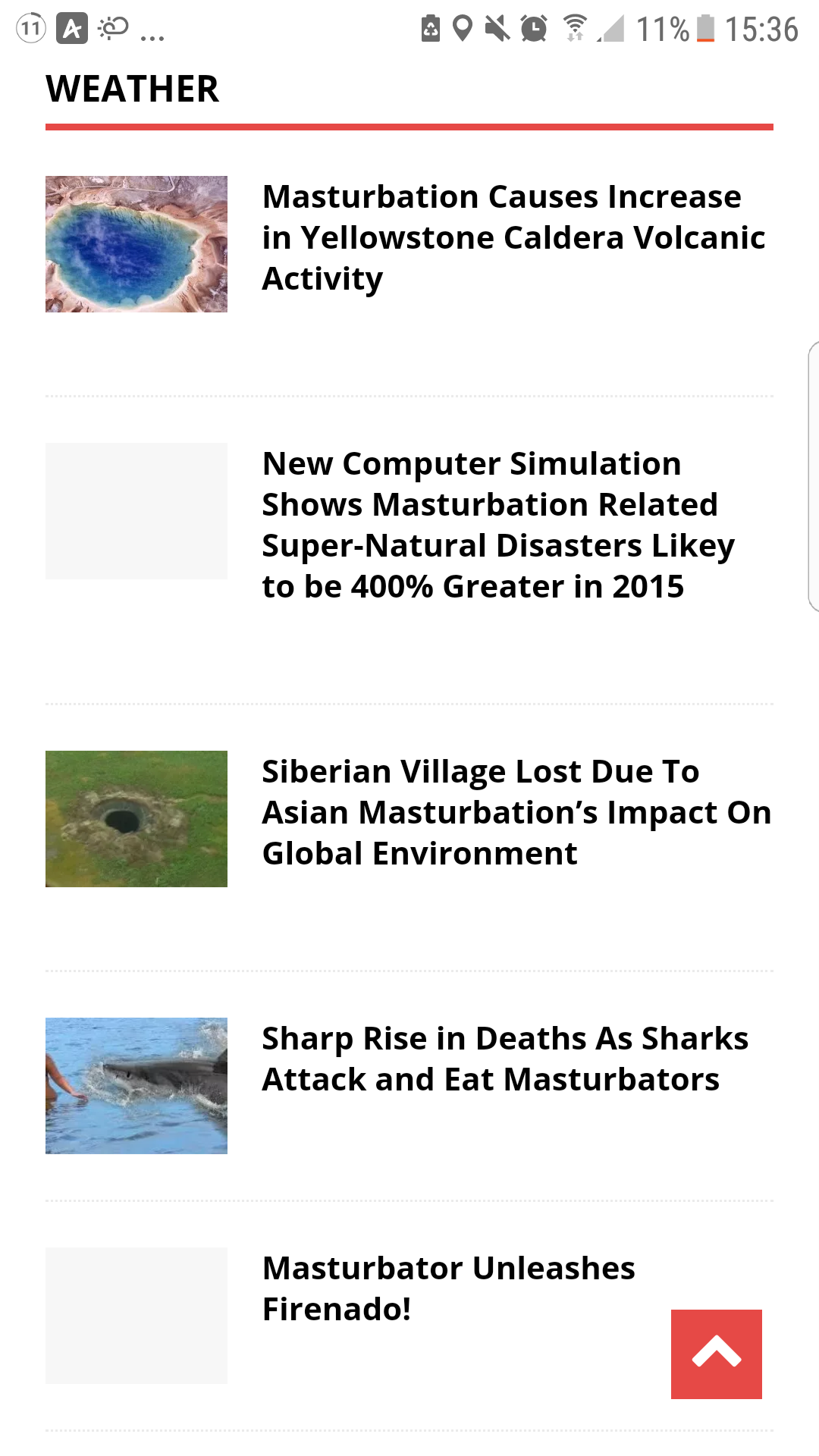The image is a screenshot of a smartphone displaying a website interface. At the top right, the current time is shown in military format as 15:36. Adjacent to the time, the battery icon is visible, filled in red to indicate a low charge at 11%. Moving left, the phone's signal strength shows only one bar, followed by a fully filled Wi-Fi signal icon. Next to these icons are an alarm clock symbol, a muted speaker icon indicating notifications are off, a location tag, and a recycling symbol.

In the top left corner, the number 11 is displayed, with a box containing the number 4 next to it. Below this, the word "Weather" is prominently displayed in black text. The main content of the page features a vertical list of article titles, each accompanied by a thumbnail image to the left. The first article includes an aerial view of a lake and bears the provocative title "Masturbation Causes Increase in Yellowstone Caldera Volcanic Activity." There are four other articles listed, with the third and fourth, as well as the first, having accompanying images.